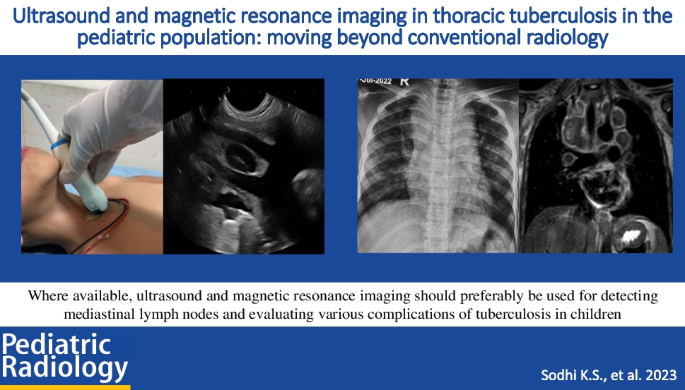This detailed image serves as an advertisement for the radiology department, particularly emphasizing advancements in pediatric radiology for diagnosing thoracic tuberculosis. Featured prominently at the top in blue text is the title: "Ultrasound and Magnetic Resonance Imaging in Thoracic Tuberculosis in the Pediatric Population: Moving Beyond Conventional Radiology." The image is framed by a blue border.

In the top left corner of the main image array, a patient lies on their back while an ultrasound wand is applied to their neck, capturing a realistic clinical moment. The other three images, positioned side-by-side to the right, depict various X-ray scans. The top two images showcase chest X-rays; the left image highlights the ribs while the right image reveals the internal thoracic structures. The third image, remaining consistent in the black-and-gray color scheme, focuses on more detailed bone structures, possibly including the spine.

Below these central images, additional text in black provides further information, likely explaining the applications and benefits of these advanced imaging techniques. The bottom left corner of the image prominently displays "Pediatric Radiology" in white text against a blue background, whereas the bottom right corner credits "SOTYKS et al, 2023." This comprehensive and visually engaging image emphasizes the role of advanced imaging techniques in improving pediatric healthcare outcomes.